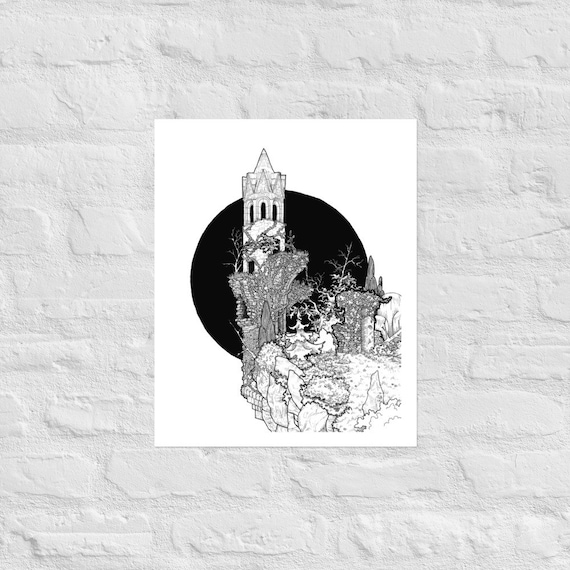This image features a detailed black and white drawing mounted on a white brick wall. The drawing is centered on a bright white sheet of paper and appears to depict a fantastical scene. At the forefront, there is an imposing tower covered in vines, with a pointed top and several windows, suggesting an old, perhaps ancient structure. The tower is perched on the edge of a cliff teeming with trees, smaller rocks, and indistinct shapes, creating a chaotic yet natural look. Behind the cliff and tower, a solid black sphere, reminiscent of either a sun or moon, dominates the sky, adding a mysterious element to the scene. The intricate details make the illustration appear hand-drawn and evoke a sense of otherworldly grandeur.